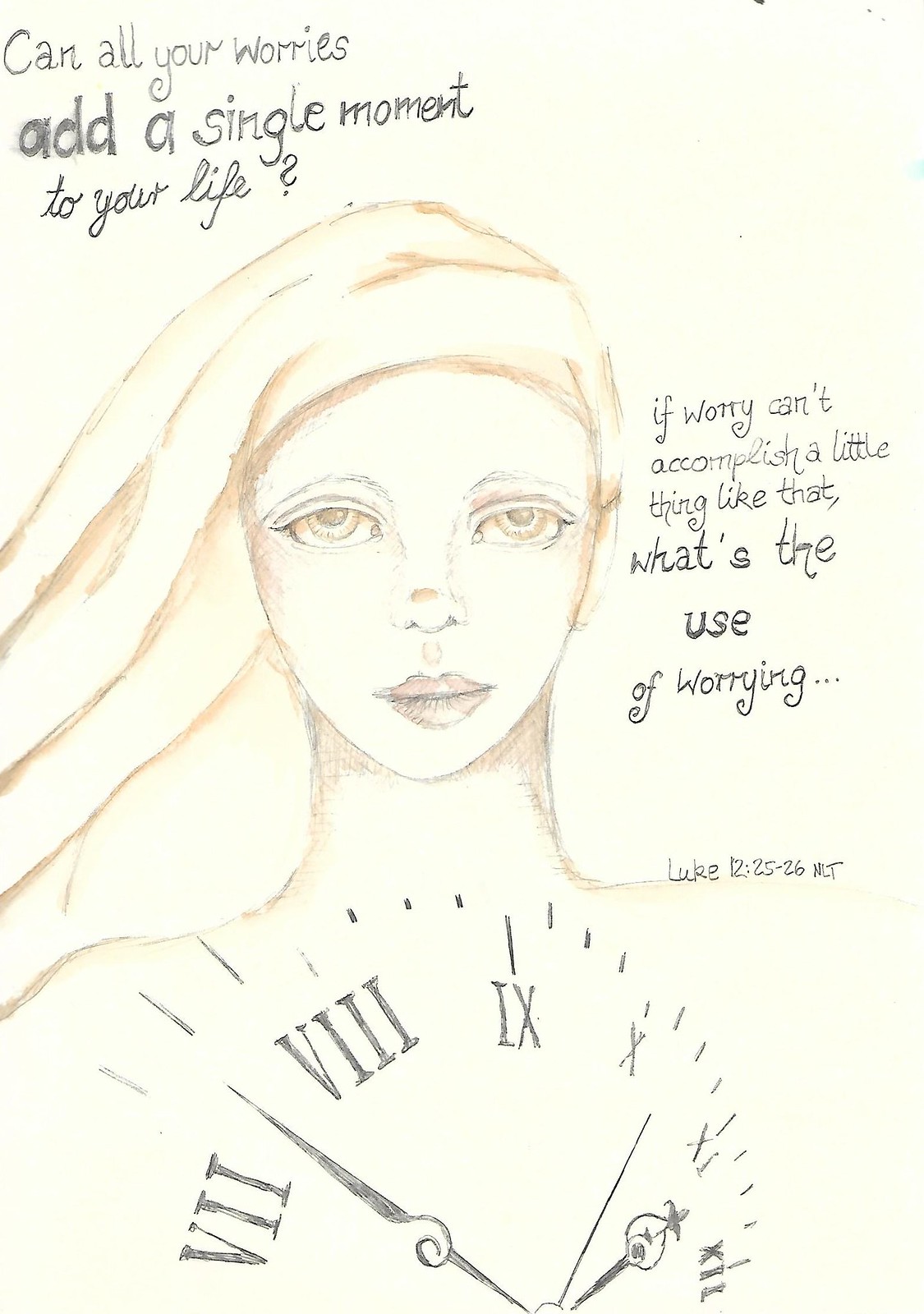The image is a detailed hand-drawn illustration of a woman located in the top left corner. She has strikingly large, yellow-tinted eyes and is looking directly at the viewer. On her head, there appears to be a long, flowing headscarf billowing off to the left side of the image. Her chest features a clock with Roman numerals. 

Surrounding the woman are several lines of text in black font. At the top of the image, the text reads: "Can all your worries add a single moment to your life?" Some of this text is written in cursive, and the question mark appears to be upside down. To the right of the woman, additional text states: "If worry can't accomplish a little thing like that, what's the use of worrying..." Finally, below this text, on the woman's right shoulder, is a citation: "Luke 12:25-26 NLT."